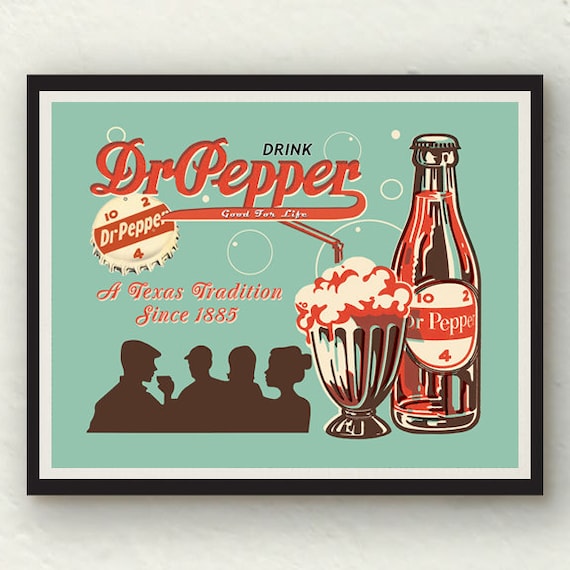This image is a detailed rendition of a classic Dr. Pepper advertisement, framed in black with a white mat, set against a white wall. The central artwork itself features a light aquamarine or mint green background adorned with thin bubbles, enhancing its nostalgic ambiance. Dominating the poster is the iconic red Dr. Pepper logo, encapsulated with the slogan "Drink Dr. Pepper" in red script above it, and "Good For Life" directly underneath. 

To the right, a meticulously drawn glass bottle of Dr. Pepper takes center stage, prominently displaying the distinctive "10, 2, 4" markings and topped with a vintage bottle cap. Beside the bottle sits a hand-drawn illustration of a frothy soda float or ice cream sundae, complete with a straw poking out, further evoking timeless soda fountain imagery.

At the bottom, the tagline "A Texas Tradition Since 1885" is smartly placed, drawing attention to the brand's long-standing heritage. Below this line, the silhouettes of four individuals can be seen, engaged in conversation and enjoying their drinks, one notably wearing a derby hat, adding a touch of period-specific charm.

Overall, this framed advertisement encapsulates the essence of a bygone era, combining visual appeal with rich historical context, making it a quintessential piece of Dr. Pepper's promotional legacy.